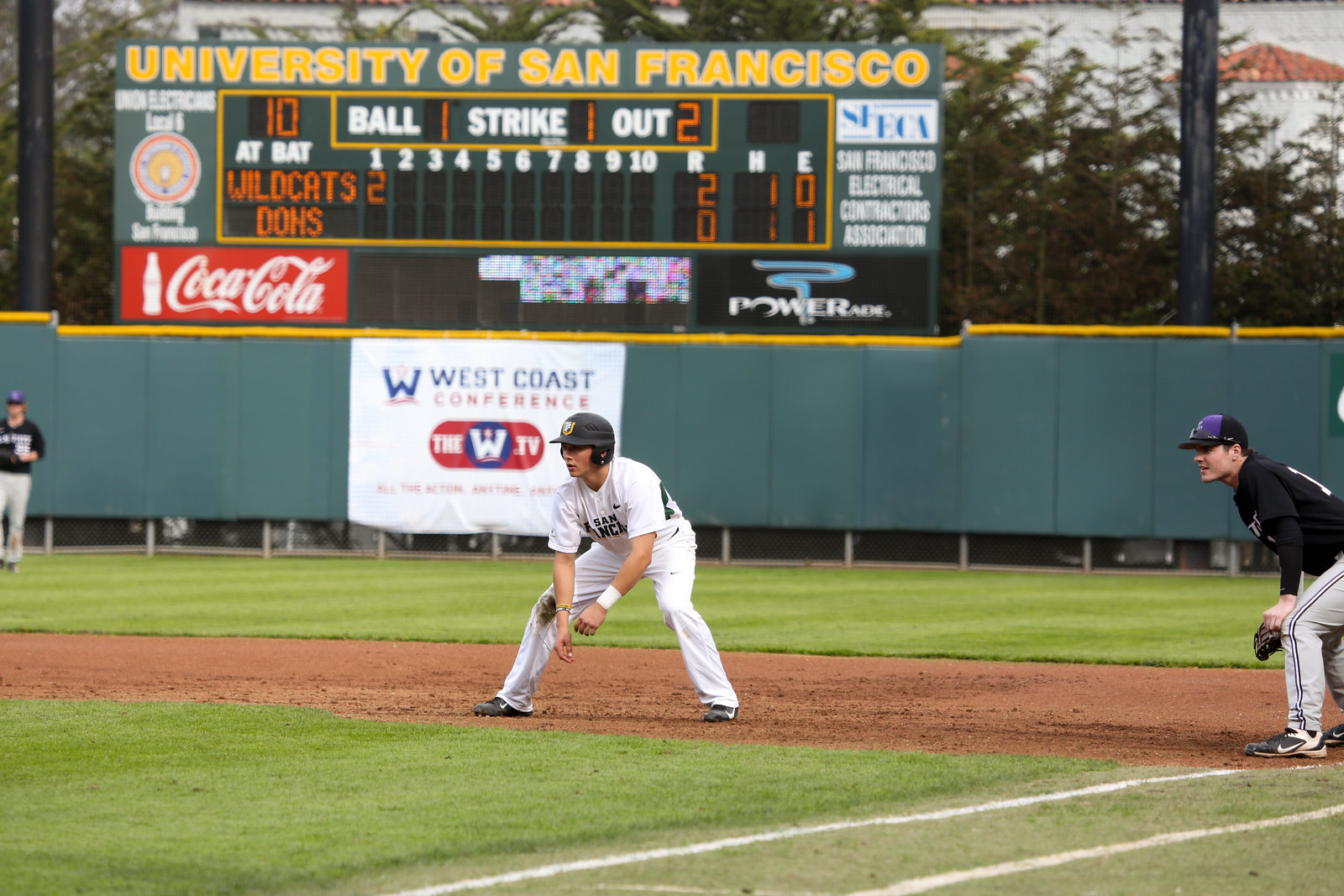In this photo taken at a baseball game at the University of San Francisco, the action is centered on a player in a white uniform, presumably a member of the home team, the Dons. This player is bent over, poised and ready for the next play, possibly anticipating a hit. Positioned nearby on first base is an opposing player from the Wildcats, identified by their black and white uniform, standing with a vigilant posture, perhaps hinting at a potential steal. Another Wildcats player is visible in the outfield to the left, also clad in black with white pants, attentively prepared for any long hits.

Prominently featured in the background, the large electric scoreboard dominates the scene with bright yellow letters proclaiming "University of San Francisco" at the top. Just below, it displays the matchup: the Dons versus the Wildcats. The scoreboard indicates that the Wildcats have scored two runs and currently have one hit, while the Dons have no runs, one hit, and one error. The game is in the bottom of the first inning with one ball, one strike, and two outs. Below the scoreboard, further details reveal advertisements for Coca-Cola and Powerade, adding a splash of color to the backdrop.

Flanking the scoreboard, a sign reads "West Coast Conference," situating the game within the collegiate sports context. Behind this setup is a picturesque grove of trees and a building peeking through, which frames the lively baseball action against a serene, natural backdrop. The well-maintained outfield grass reflects the readiness and care put into the field, highlighting the excitement and anticipation that comes with competitive baseball.